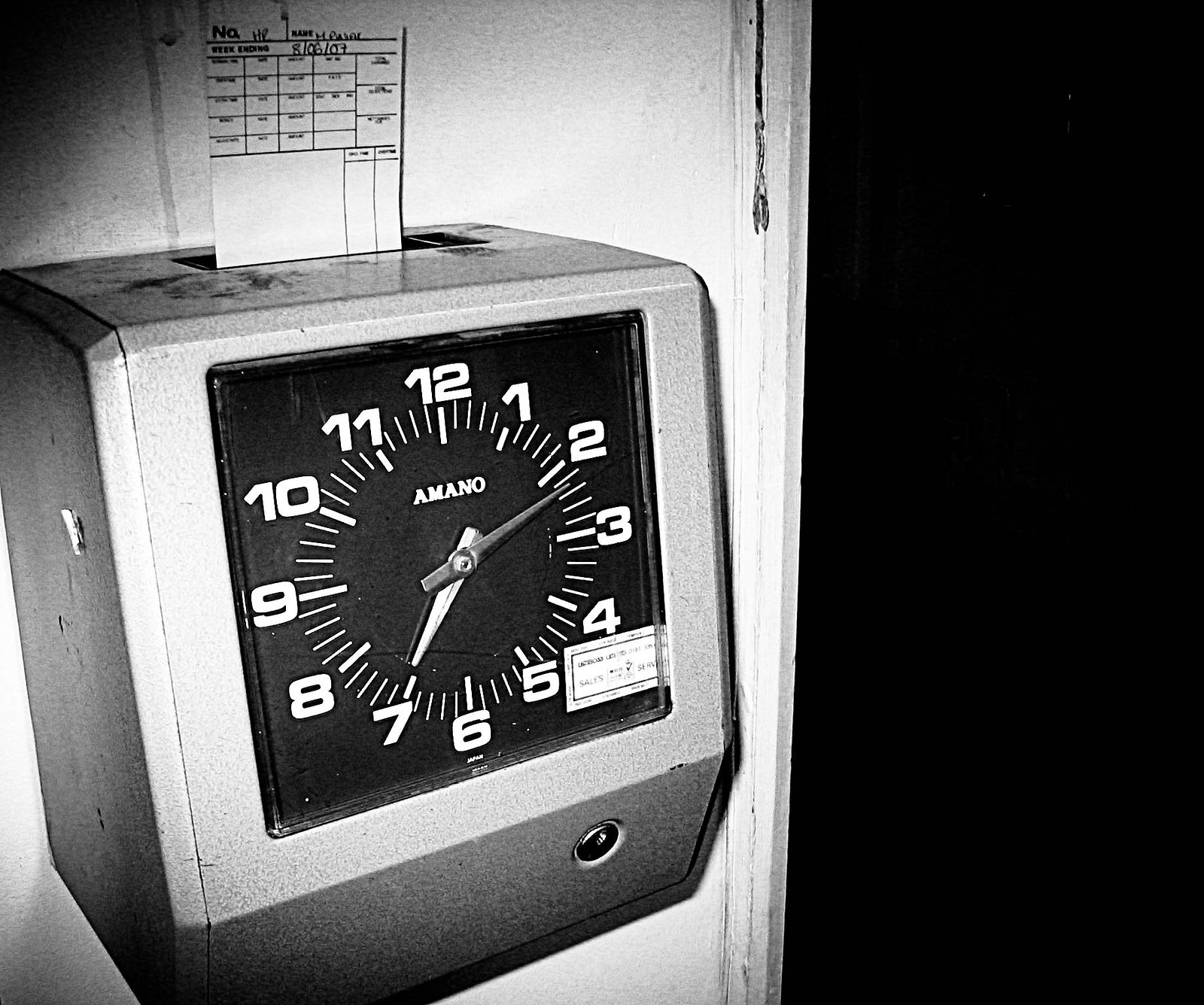This black and white photograph features a stark contrast, with the right side entirely in black, creating a dramatic backdrop. On the left side, a pristine white wall serves as a canvas for a prominent focal point: a vintage time clock. The time clock is square in shape and appears to be constructed from metal, suggesting durability and industrial use. Its front panel displays a black square face with clearly marked white hours and the name "Amano" positioned just below the number 12. The clock's hands are set to 7:11, indicating the current time. Below the clock face, a small circular keyhole is visible, hinting at a mechanical aspect that requires a key for access. At the very top of the time clock, a slot is present, holding a piece of paper, suggesting an action akin to clocking in or out. The composition and tones create a captivating historical narrative of workplace routines.